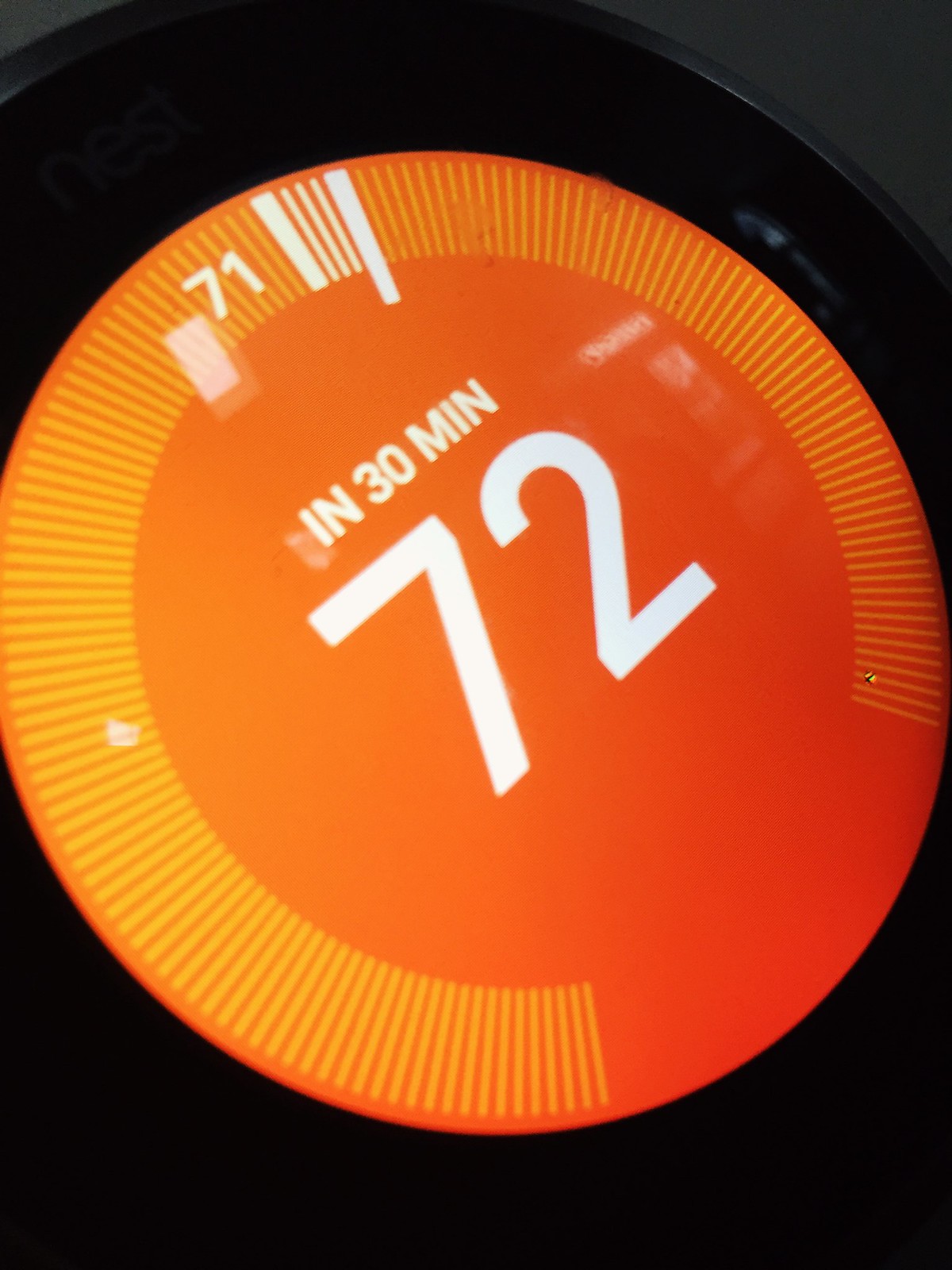A high-resolution photograph captures a sleek, black, round digital thermostat prominently displayed against a neutral background. The thermostat features a central digital display with modern aesthetics, predominantly showcasing shades of dark and light orange. Reflections of ambient light are subtly visible on its surface, adding a touch of realism to the image. 

In the center of the display, the temperature reads "72" in bold white font, with a smaller text above it stating "in 30 minutes." The display is further accented by a series of orange dashed lines that encircle the upper half of the thermostat. At the top of the display, the current temperature "71" is indicated in white font, complemented by white dashed lines alongside varying hues of white to orange lines that form a circular pattern around the screen.

The photograph is devoid of any additional objects, focusing solely on the thermostat, and the image quality is notably clear, allowing for a detailed view of the intricate display and design features of the device.